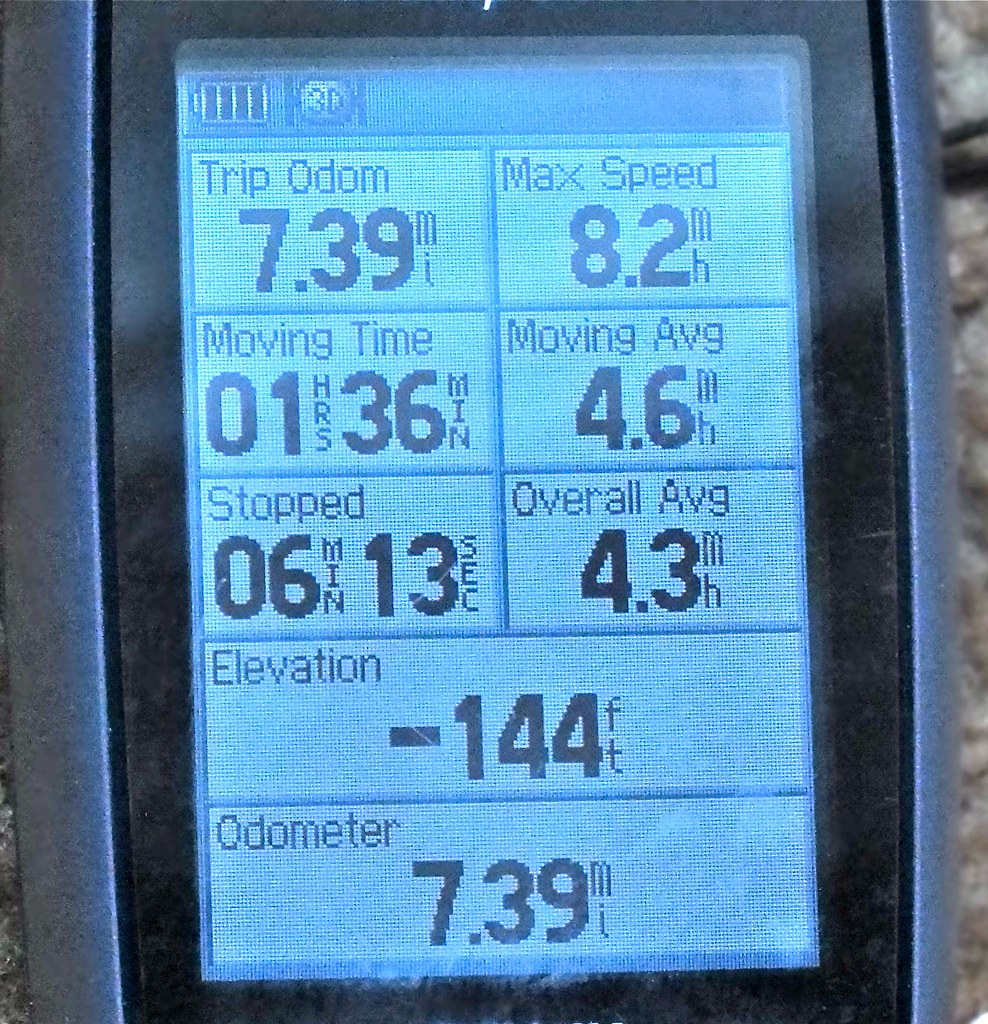The image displays a screen with a gray border and a black outline. In the top left corner of the screen, there is a battery icon indicating full charge. Below the battery icon, the trip odometer reads 7.39 miles. To the right, the maximum speed is shown as 8.2 miles per hour. On the left side, the moving time is displayed as 1 hour and 36 minutes with a moving average speed of 4.6 miles per hour. Below that, the stopped time is listed as 6 minutes and 13 seconds, with an overall average speed of 4.3 miles per hour. At the bottom, the elevation is noted as negative 144 feet, and the odometer shows a total of 7.39 miles.